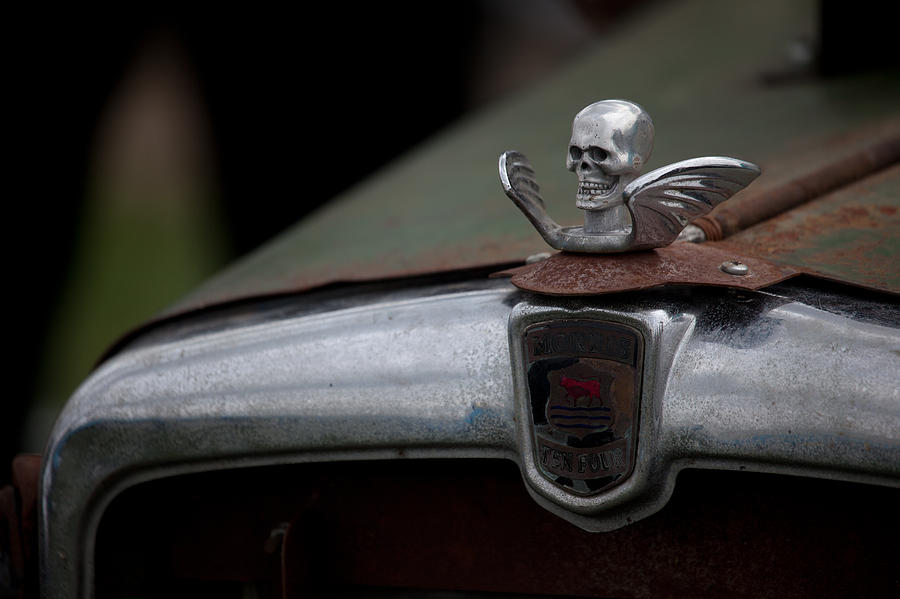In this photograph, the focus is on the hood of a very old, rusty vehicle—potentially a truck or a military vehicle. The hood ornament is a striking, novelty design featuring a skull with bat wings, crafted out of what appears to be chrome or silver. This ornament is affixed to the heavily patinaed hood, which exhibits a matte, flat finish with significant rust and water spots, adding to its vintage character. The background of the image is blurred, keeping the attention on the front end of the car, which includes a partial view of the grill and an indistinct, possibly military-looking emblem. Despite the poor lighting and less-than-crisp details, the ornament's retro goth aesthetic and the vehicle's overall state lend a spooky, nostalgic vibe to the scene.